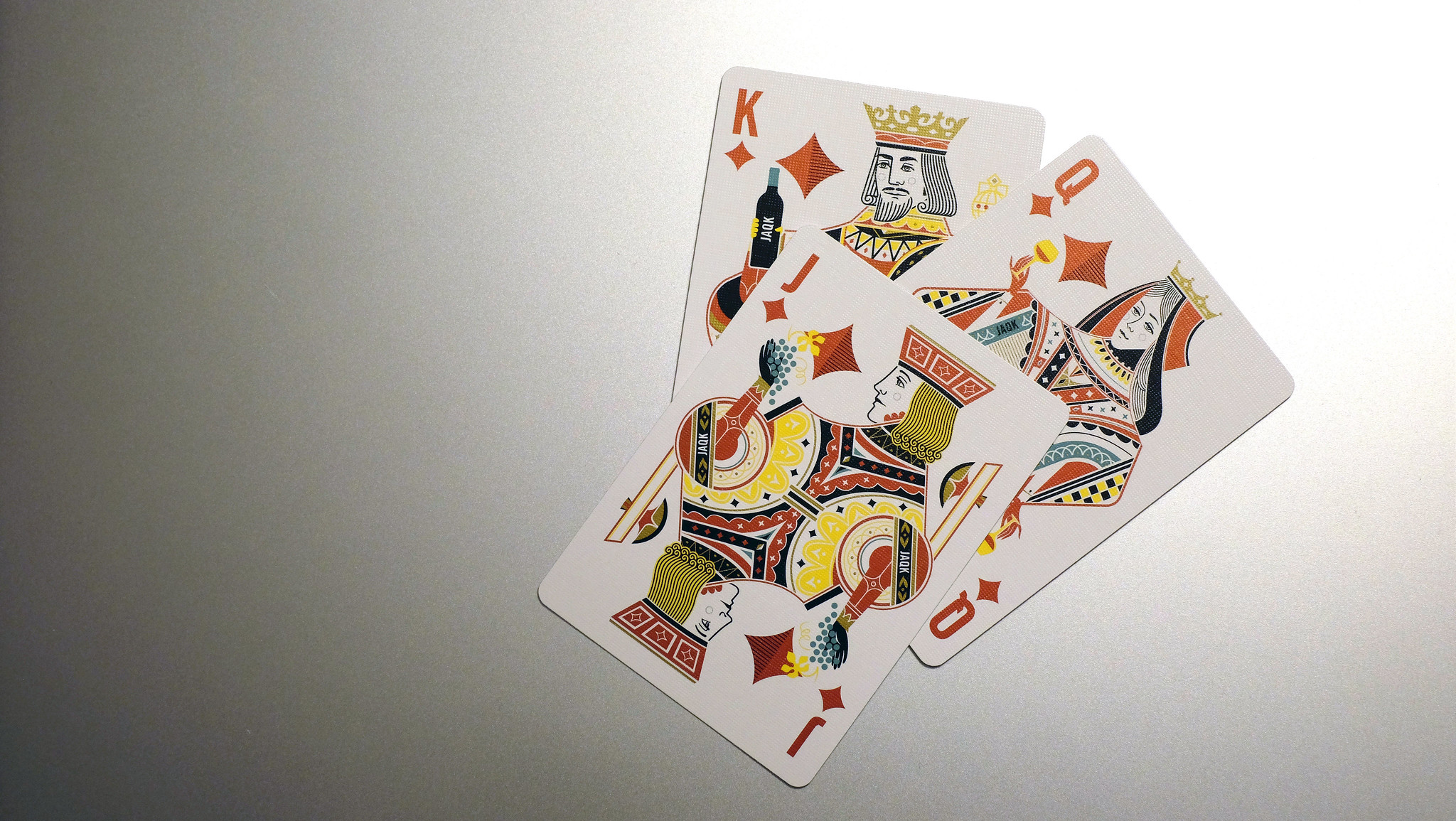The image features a gradient background that transitions smoothly from dark gray on the left to almost white on the right. Positioned towards the right side of this gradient is a slightly fanned-out stack of three playing cards, specifically from the Diamonds suit, each showcasing intricate designs.

At the top of the stack is the Jack of Diamonds, depicted with blonde hair and wearing a crown. He is defiantly holding a sword, symbolizing his readiness and valor. Below him is the Queen of Diamonds, adorned with a crown matched with a red veil. She has long gray hair and is dressed in luxurious robes, embodying elegance and authority. At the bottom of the stack is the King of Diamonds, who stands out with his elaborate crown. He has a distinguished beard, mustache, thick eyebrows, and long gray hair. The King is holding what appears to be a bottle of wine, reinforcing his royal and opulent presence.

Each card is detailed with the red suit's characteristic diamonds, further enhancing the regal and thematic unity of the group.